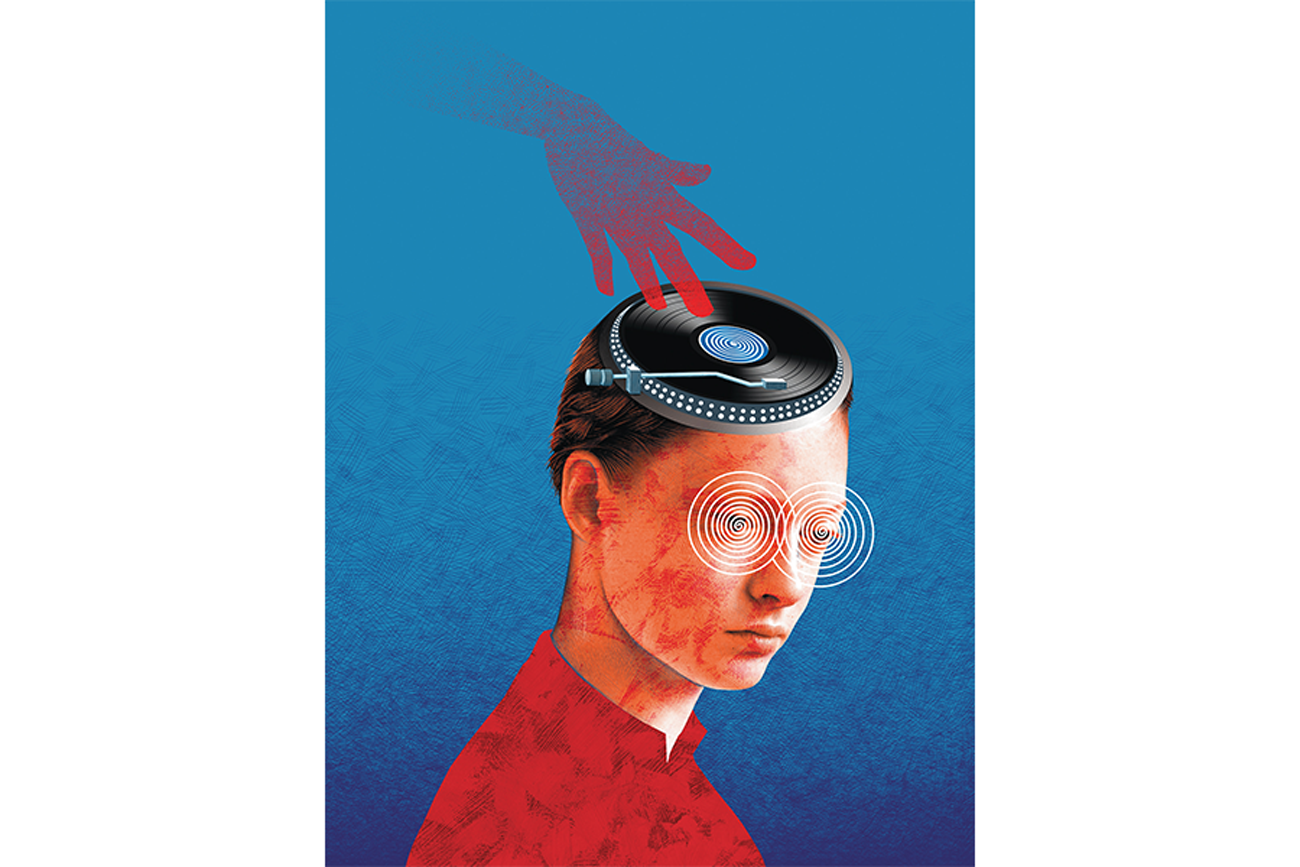The image depicts a young man, reminiscent of a teenage Macaulay Culkin, set against a textured blue background. The man, who sports slicked-back brown hair and an androgynous appearance, wears a red shirt with a brush-textured pattern. His eyes are adorned with hypnotic spiral circles, adding to the surreal feel of the image. Distinct blotchy red patches appear on the sides of his face, which could be interpreted as blood splotches. Atop his head rests a DJ turntable, fashioned like a small cap, with a record that is black with a blue center label. From the top left of the image, a hand, graduated in color from blue to purple to red fingers, descends to spin the record, mimicking the actions of a DJ. The background transitions in a gradient of blue and purple hues, enhancing the overall ethereal and odd style of this AI-generated artwork.